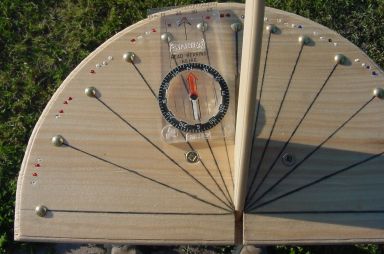The photo depicts a wooden half-circle sundial positioned outdoors on a patch of grass. The sundial features an arch with red and white rivets or domed screws around its outer edge, each with black lines radiating towards the center, creating a pattern similar to a speedometer. Sunlight illuminates the sundial, highlighting its intricate design. At the top-left section of the sundial, a transparent compass is placed, oriented towards the north, adding to the sundial's detailed setup. The sundial appears to be supported by a vertical wooden post, further enhancing its sundial effect.